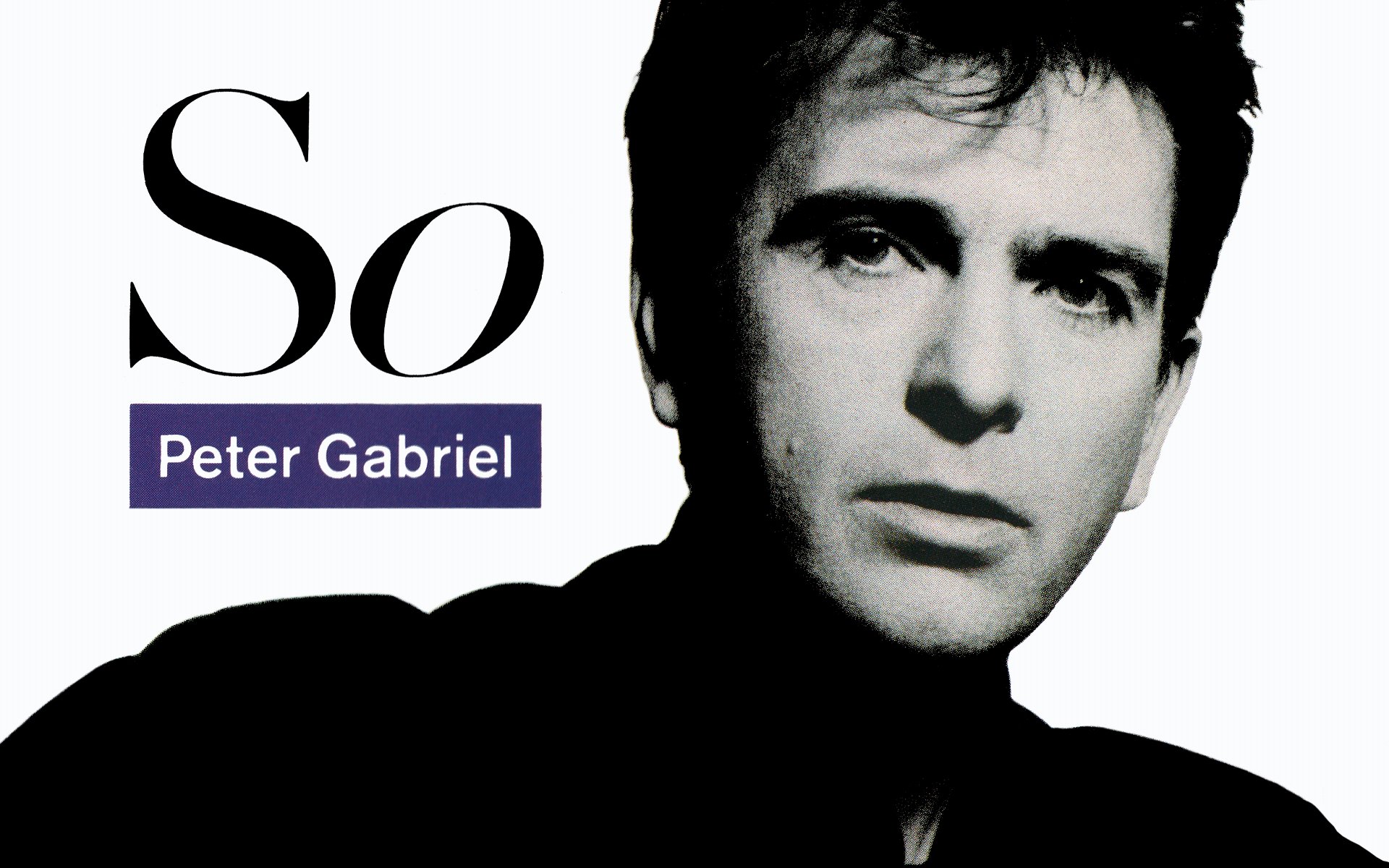This black-and-white photograph features the cover of Peter Gabriel's album "So." Dominating the top left corner is the album's title, "So," rendered in large black text. Directly beneath this, within a small blue rectangle, are the words "Peter Gabriel" in smaller white letters. The background is a stark, uninterrupted white, contrasting sharply with the central portrait of Peter Gabriel himself. The image captures Gabriel from the neck up, his face partially obscured by heavy shadows, which lend a dramatic effect to the cover. He appears to be wearing a black top, potentially a turtleneck, although the shadows make it difficult to discern precise details. Gabriel’s hair is dark and short, with a slight dishevelment as a lock falls over his forehead. He has a neutral expression with a slight gaze to the left, his thick eyebrows adding to his intense look. Notably, there is a small mole visible on his left cheek.